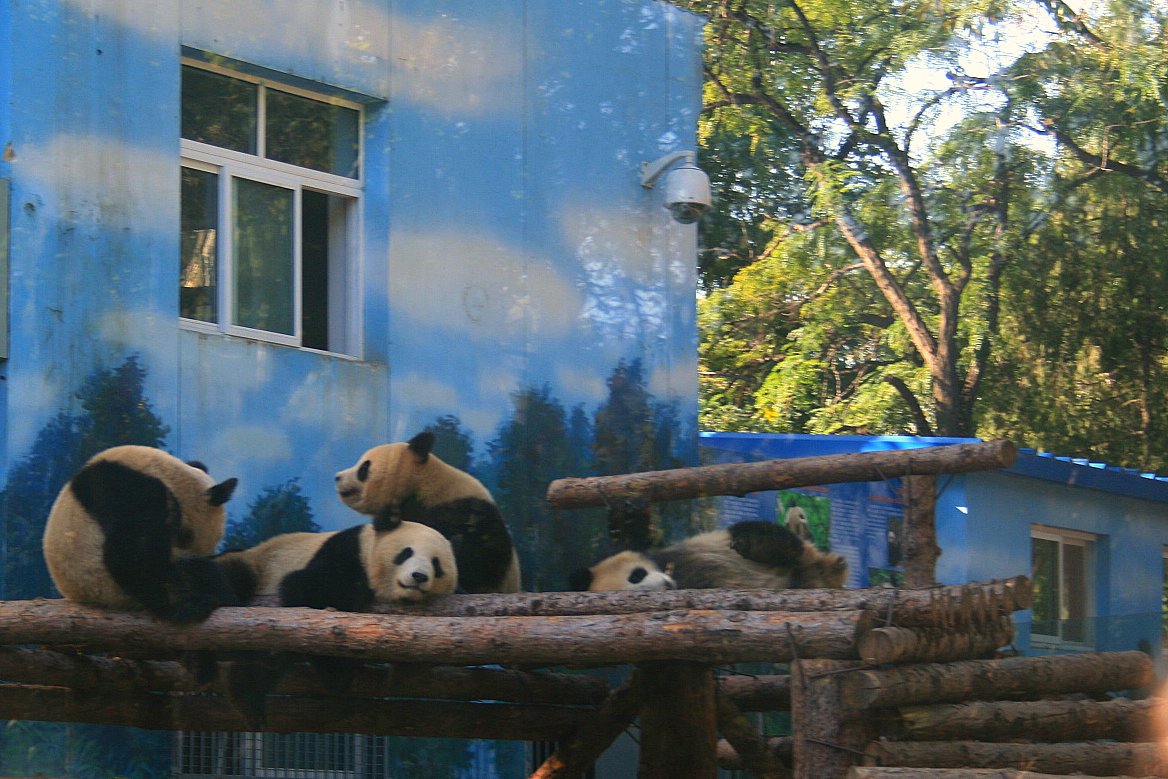In this outdoor color photograph, a group of panda bears occupies the center and lower portion of the image, likely within a zoo or sanctuary habitat. At the heart of the scene is a horizontally cut log structure that the pandas are lounging on. The panda bears, with their distinctive black-and-white markings, are variously positioned—one hunched over facing right, another appearing to sleep with its head down, and one peeking over a rock. Notably, a curious long-haired panda distinguishes itself among the group.

Behind these pandas, a large building painted light blue serves as a backdrop. This building features a mural depicting trees and clouds, enhancing the scene's outdoor ambiance. A centrally-located open window and a visible webcam or monitoring device protruding from the wall add functional elements to the setting. To the right, fully grown green trees provide natural context, and a smaller, similarly painted shed near the bottom right corner completes the setting. No text or signage is visible in the image, emphasizing the serene environment of the pandas’ enclosure.